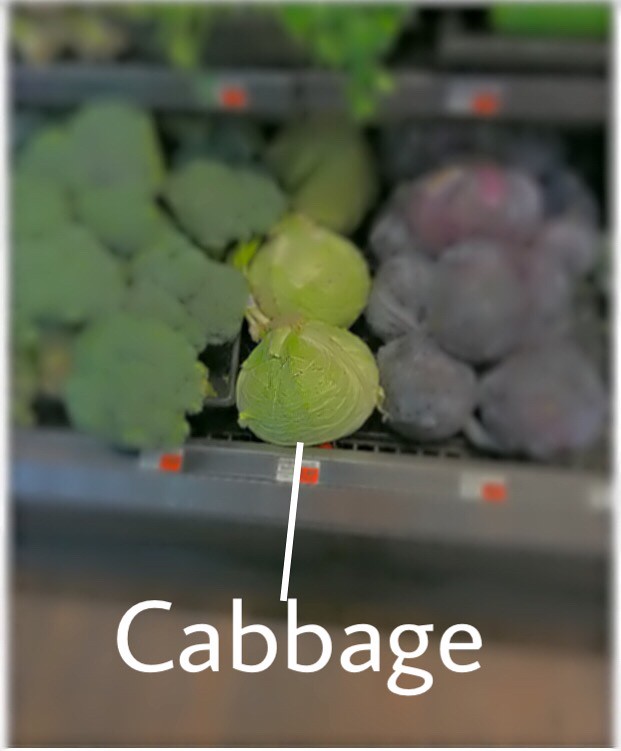The photograph captures the produce section of a grocery store, focusing primarily on a tiered shelf of vegetables. The image quality is notably poor, with most items appearing blurred, except for a few distinct heads of green cabbage. In the center, three green cabbages are clearly displayed in a row, accompanied by a white line connecting to the word "cabbage" in white text at the bottom of the image. Surrounding these cabbages, on the left side, there are florets of broccoli, and on the right, what appear to be heads of red cabbage, though both are heavily blurred. Each vegetable grouping has price labels, characterized by white tags with small orange stickers. Above this bottom shelf, there's another shelf holding various green vegetables, all blurred, making it difficult to identify specific types. The entire setting is presented on flat gray shelving, reinforcing the focus on the clear cabbages in the center amidst the overall blur.